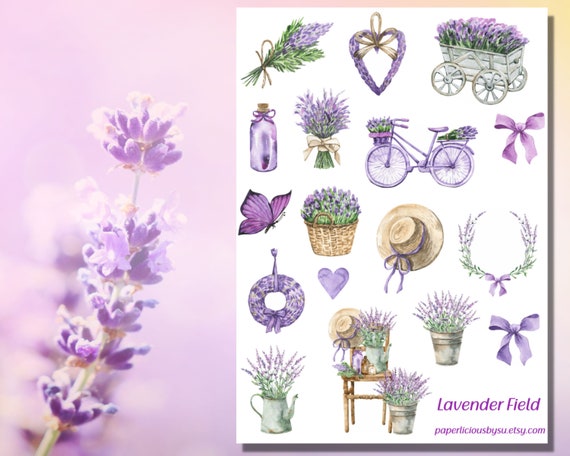The image features a stunning close-up of a lavender flower cluster on the left, set against a subtly pink-lavender blurred background. This photograph occupies about 40% of the image and showcases the delicate purple blossoms at multiple levels along the stem. The remaining 60% of the image to the right displays a detailed, intricately drawn advertisement for an Etsy shop, "paperliciousbysu.etsy.com," titled "Lavender Field." Within this drawing, various charming lavender-themed decor items are meticulously illustrated: a bundle of dried lavender, a heart-shaped lavender wreath, a cart brimming with lavender, a lavender-colored bottle adorned with a bow and cork, a purple bicycle with lavender-filled baskets, several decorative purple bows, a lavender butterfly, a straw hat accented with a lavender ribbon, numerous planters with lavender, and a chair hosting these items. The collage reveals an assortment of creative uses for lavender, emphasizing its decorative and aromatic potential in a harmonious purple palette.